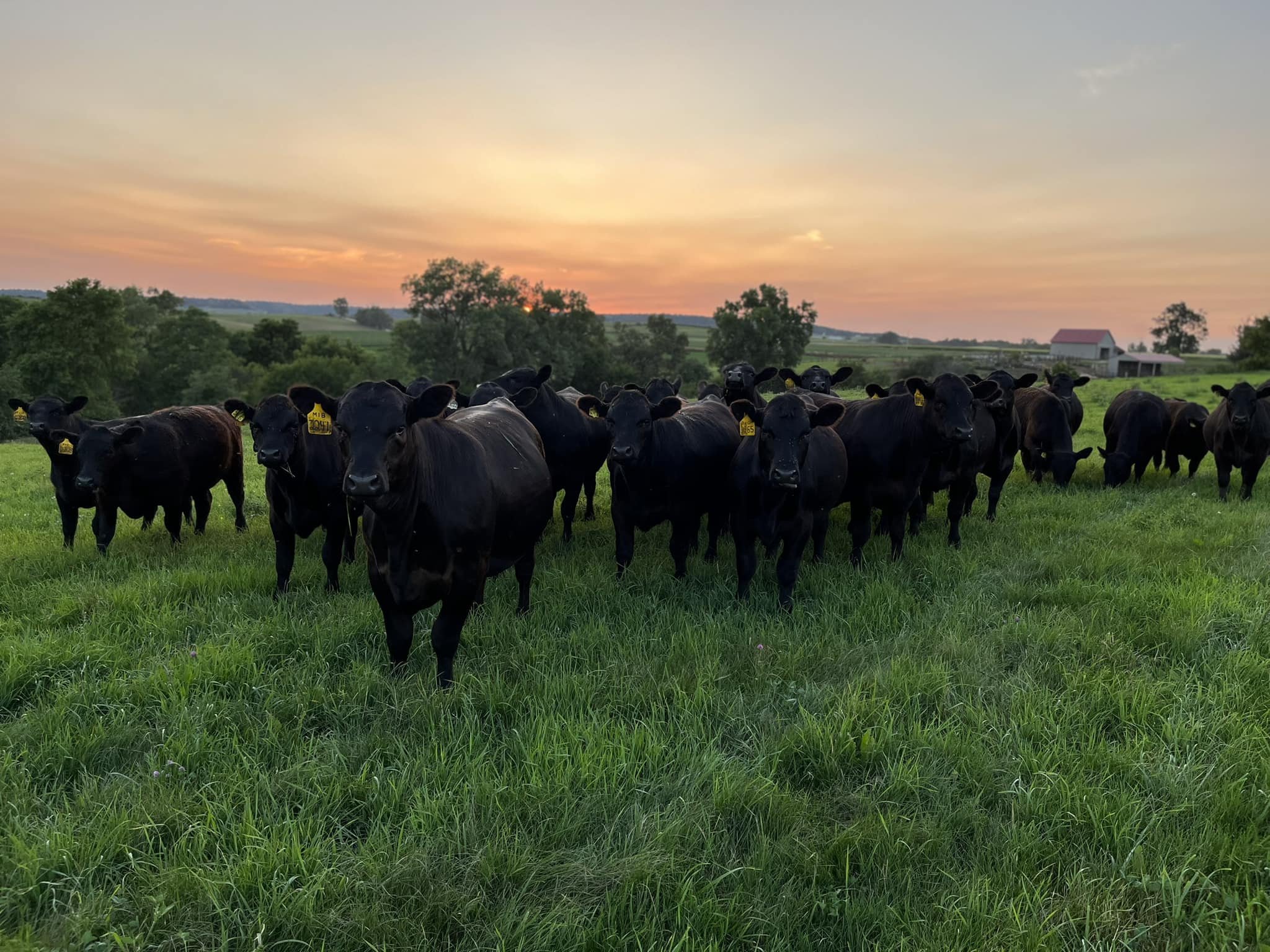In this detailed outdoor photograph, a lush green pasture is populated by a herd of over a dozen black cows, with each cow sporting a bright yellow identification tag on its left ear. The animals are positioned at varying distances from the camera, with some standing only a few feet away while others are dispersed across the mid-ground and background. Several of the cows are grazing, while a few are attentively staring towards the camera. The picturesque scene is captured during either the early morning or the late evening, signified by a beautiful yellowish-reddish hue from the setting or rising sun in the distance, casting a soft glow over the landscape. The sky above transitions from warm tones to a cooler gray-blue. In the background, there are also some trees, buildings, and barns set against a gentle hill, enriching the pastoral atmosphere of this serene countryside moment.